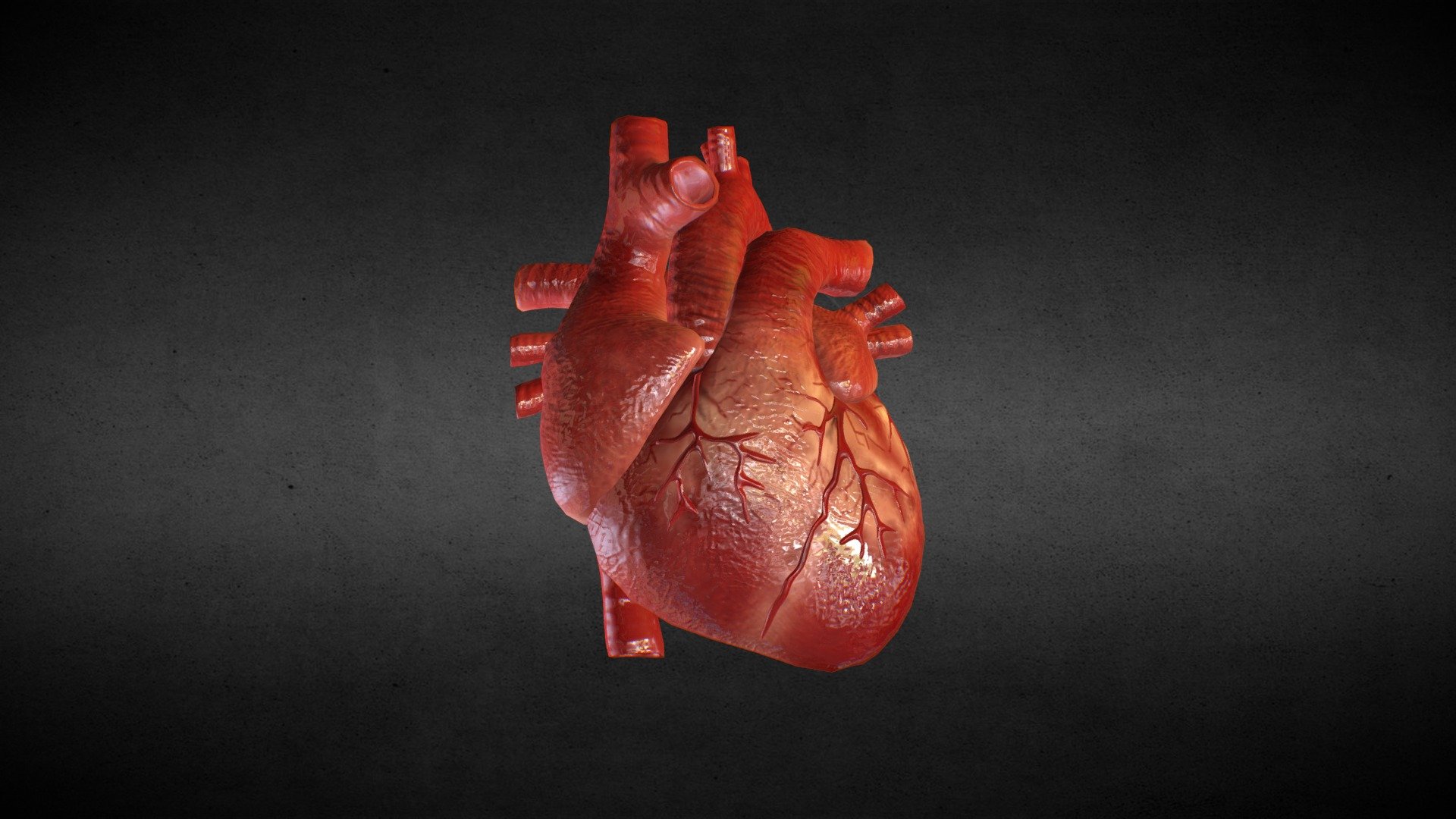The image features a three-dimensional rendering of a human heart, positioned prominently in the center of the frame. The heart is predominantly a deep red color, with areas exhibiting yellowish or orangish tints. Veins and arteries are visible, particularly around the largest chamber, adding to the overall detail of the depiction. Several tubes, likely representing major blood vessels, extend from the top, sides, and bottom of the heart.

The background is black, with a horizontal band across the middle that appears slightly lighter, suggesting a reflection or shadow. The rectangular image is bright and clear, with sufficient lighting that enhances the depth and detail of the heart, giving it an almost realistic, three-dimensional appearance. The image features no additional elements, such as text, numbers, or other distractions, allowing full focus on the heart.